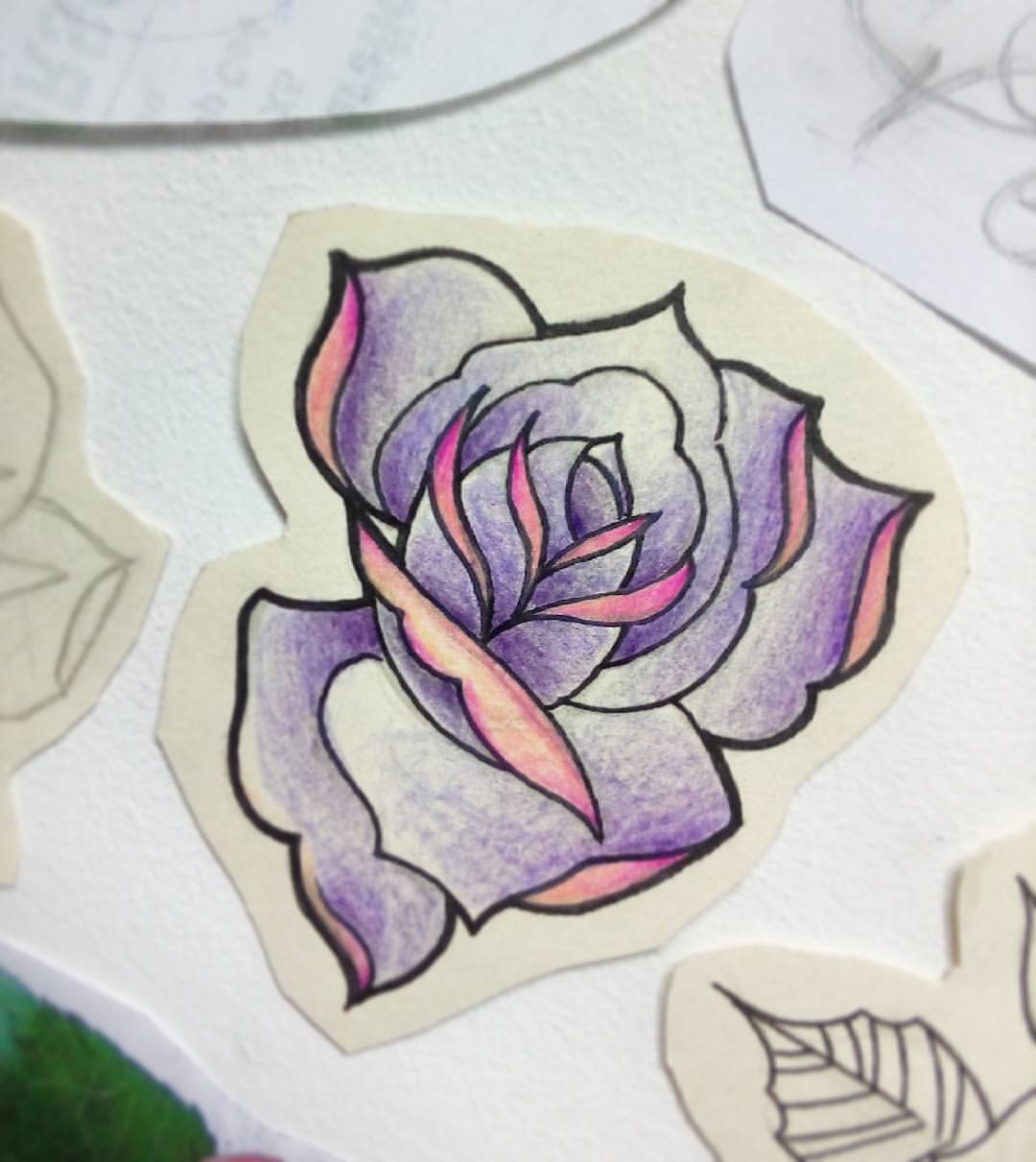This photograph features a collection of intricately cut-out art pieces displayed against a white background. At the center of the image, there is a striking flower with vibrantly shaded petals, showcasing a gradient from pink at the interior to a mix of purple and white at the edges, suggestive of detailed colored pencil work. The petals' contours are outlined in black ink, enhancing the depth and precision of the flower's appearance. Surrounding this central flower are other partially visible cut-outs, each bordered in a tan color, giving them a sticker-like quality despite being paper artworks. Notably, in the bottom right corner, there is another cut-out featuring a simple black and white leaf drawing. Additional elements include various shaped pieces of paper—some casting subtle shadows—adding layers to the composition. In the bottom left corner, there is a faintly visible spongy green object, adding a touch of mystery to the otherwise meticulously arranged artistic presentation.